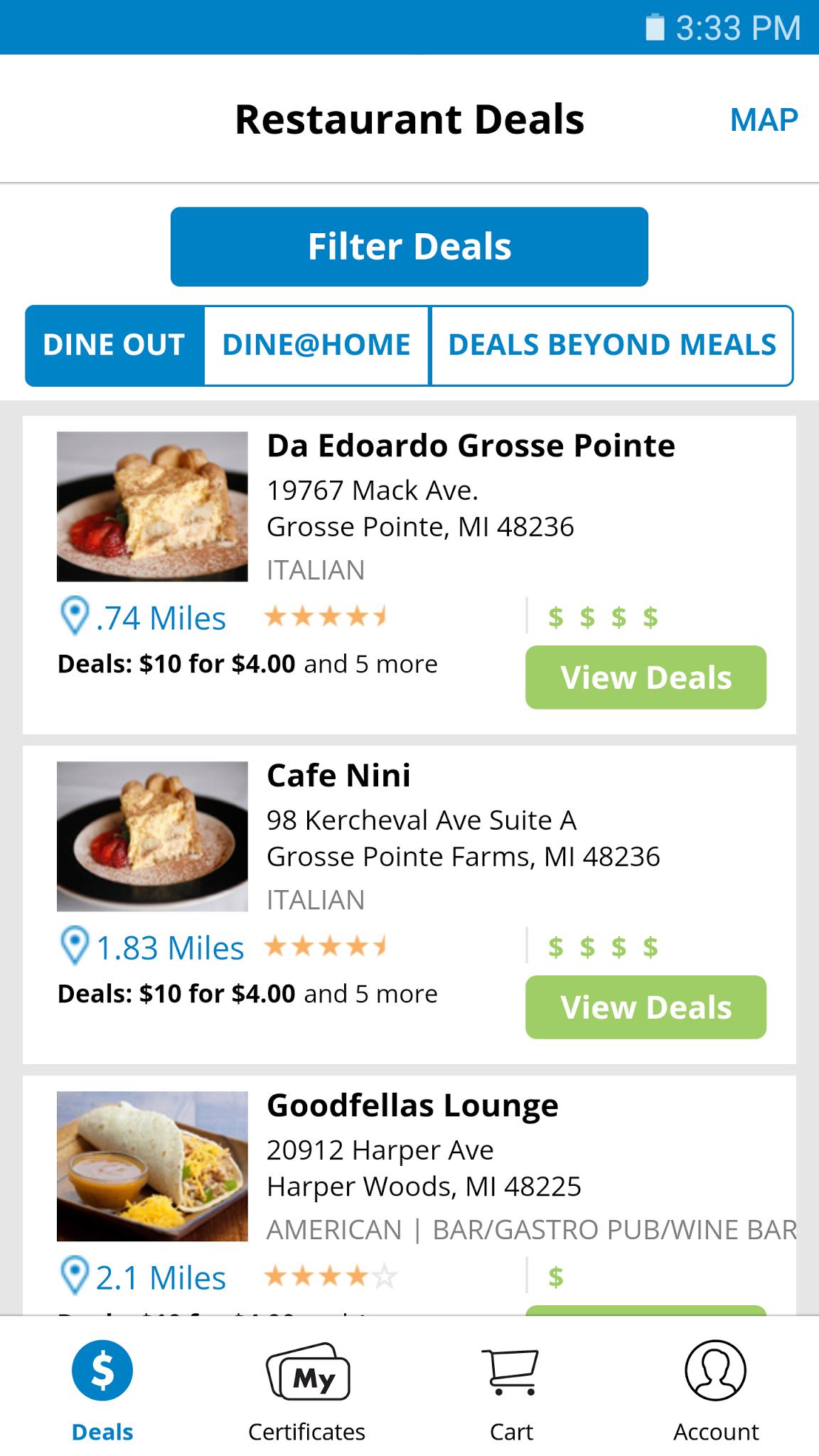This screenshot captures a smartphone display of a deals webpage with a blue border. The battery icon indicates full charge, and the timestamp shows 3:33 PM. Below that, you'll find a white "Restaurant Deals" text next to a blue "Map" button. Further down, there are buttons labeled "Filter Deals," "Dine Out," "Dine at Home," and "Deals Beyond Meals."

The page features four entries for local restaurants:

1. **D'Eduardo Grosse Pointe**  
   - **Address:** 19767 Mack Avenue, Grosse Pointe, Michigan 48236  
   - **Cuisine:** Italian  
   - **Distance:** 0.74 miles  
   - **Deals:** $10 for $4 and five more deals available  
   - **Rating:** 4.5 stars  
   - **Icon:** Dollar sign  
   - **Button:** Lime-colored "View Deals" button
   - **Image:** Slice of pie

2. **Cafe Nini**  
   - **Address:** 98 Kirstenville Avenue, Suite A, Grosse Pointe Farms, Michigan 48236  
   - **Cuisine:** Italian  
   - **Distance:** 1.83 miles  
   - **Deals:** $10 for $4 and five more deals available  
   - **Rating:** 4.5 stars  
   - **Icon:** Dollar sign  
   - **Button:** Lime-colored "View Deals" button
   - **Image:** Slice of pie

3. **Goodfellas Lounge**  
   - **Address:** 20912 Harper Avenue, Harper Woods, Michigan 48225  
   - **Cuisine:** American Bar / Gastropub / Wine Bar  
   - **Distance:** 2.1 miles  
   - **Deals:** Listed, the rest cut off  
   - **Rating:** 4 stars  
   - **Icon:** Lime dollar sign  
   - **Button:** Lime-colored button (cut off in the screenshot)

4. **Additional Entries:** Information not fully visible in the screenshot

At the very bottom of the screen, a highlighted blue bubble with a dollar sign says "Deals." To its right are icons and text for "My Certificates," "Cart," and "Account" with a user profile icon.